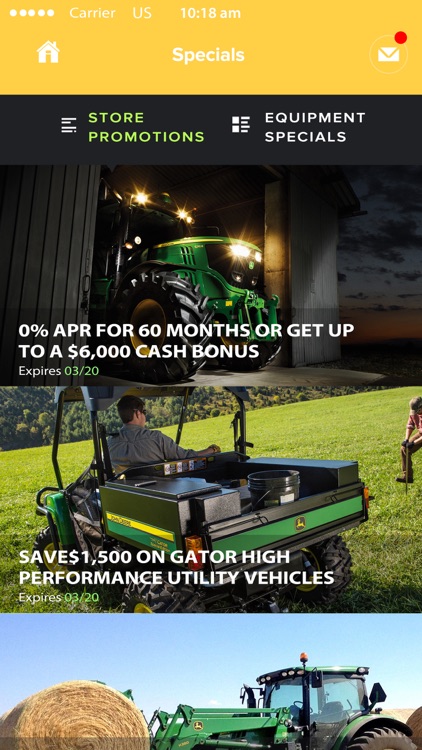A detailed and clear description for the screenshot image:

The entire screenshot is taken from a phone. The top inch and a half of the image features a dingy yellowish-gold background. On the top left corner, there are five white dots, immediately followed by the word "Carrier" in white, and then "U.S." Still in white, the center of the top section displays the time "10:18," and just below this, it reads "Specials." To the left of the "Specials" text, there is a white home icon, and on the right side, there is a white mail icon with a red dot above it.

Below this top section, there is an inch wide black border. Following that, there is a green header that reads "STORE PROMOTIONS" in all capital letters. To the left of this header are four horizontal gray lines, and next to them on the left are four horizontal white lines. The text "Equipment Specials" is written in white next to another series of lines.

Beneath this header, there is a picture of a green tractor emerging from a gray building. The tractor has lights and large black tires. Bold white text across the bottom of this picture states, "0% APR for 60 months or get up," followed by the next line, "to a $6,000 cashback, cash bonus." Below, in smaller white lettering, it says "Expires," followed by the date "03-20" in green.

Continuing downward, there is a guy sitting outside on a green and black cart with a roof. You only see his back and a nice green lawn in the background. To the bottom left, "Save $1,500 on Gator High" is bolded in white, followed by "Performance Utility Vehicles" in smaller white text. Below, in small white letters, it says "Expires" in green followed by "03-20."

The bottom picture is cut off, showing only half of a roller bale of hay, the sky, and part of a green tractor. The green section is in the center, with the cab where the person sits visible on the right side of the image.